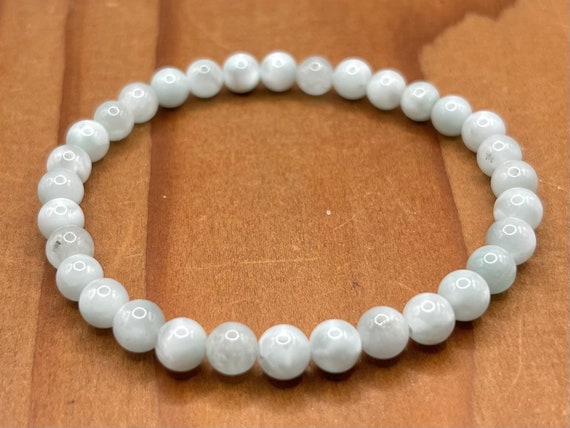This photograph showcases a necklace composed of smooth, white pearl-like beads, lying gracefully on a medium-stained wooden table. The table features a tan color with darker brown streaks that create a striking contrast. The surface highlights the natural variations in the wood, accentuated by a clear coat that enhances its grain and texture. The beads exhibit subtle transitions of color, with hints of light gray that emerge under specific lighting, adding depth to their appearance. There is no clasp visible, implying the necklace is a continuous strand. Slight reflections and the natural inclusions within the beads add to their charm, while faint marks and scratches on the wooden surface suggest its well-worn authenticity.